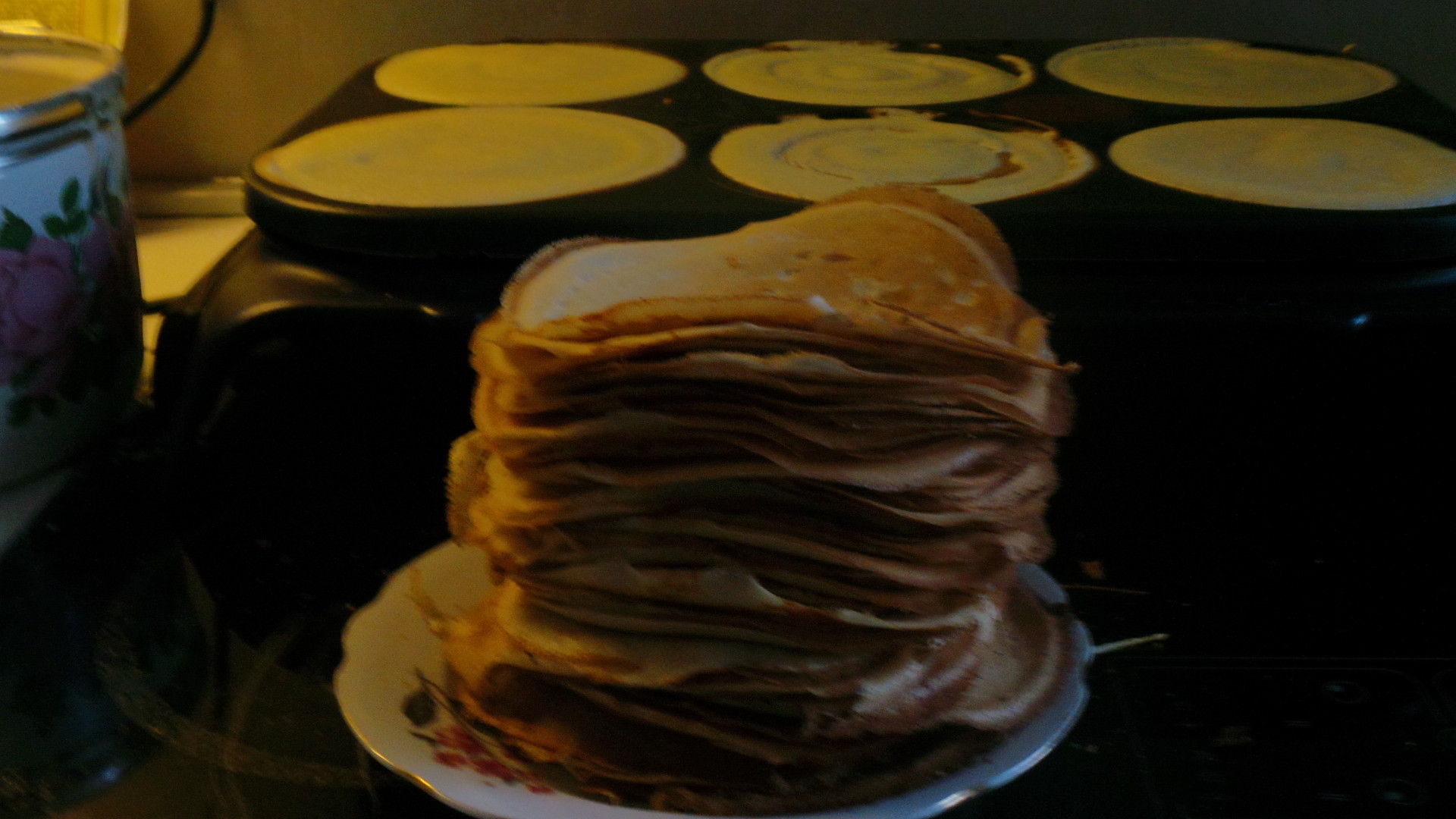This blurry photo, taken inside a home, captures a culinary scene centered around a stack of thin, crepe-like pancakes on a decorative white plate with a scalloped edge, a gold rim, and a floral pattern. The plate, laden with two or three dozen golden-brown, flaky pancakes, occupies the foreground of the image. In the background, seated on a black stovetop, six more pancakes cook on a griddle, arranged in two rows of three. These in-progress pancakes, still pale and yellow, await flipping. Adding to the homey setting, a small floral canister is visible on the far right, while a floral bowl or kettle makes an appearance on the left side.